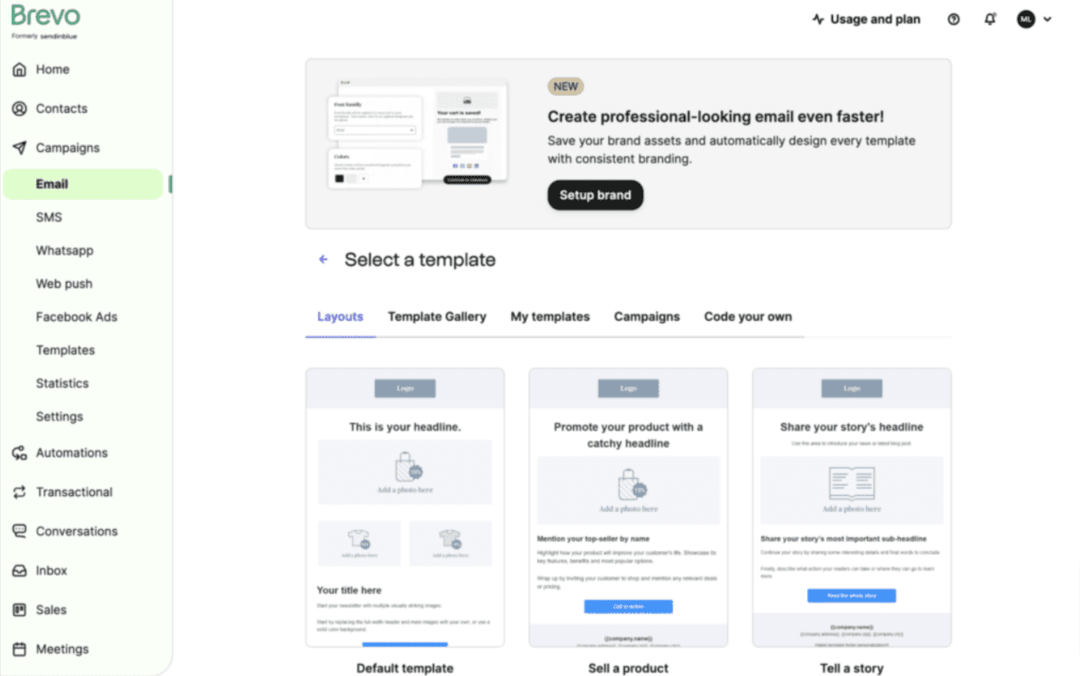The image depicts a detailed interface of the email marketing platform, Brevo. The left-hand side features a green column listing various navigational options such as Home, Contacts, Campaigns, Email, SMS, WhatsApp, Web Push, Facebook Ads, Templates, Statistics, Settings, Automations, Transactional, Conversations, Inbox, Sales, and Meetings.

On the main website screen, a gray box with large black text prominently announces, "Create professional-looking emails even faster." Below this message, it explains how users can save their brand assets and automatically design every template with consistent branding. A button labeled "Set Up Your Brand" invites users to take action. To the left of this text, an illustrative image guides users on setting up their brand, showing a piece of paper and an inset prompting template selection.

Further below, users can choose different layout options such as Layouts, Template Gallery, My Templates, Campaigns, or Code Your Own. The Layouts tab is highlighted in blue. Users are encouraged to promote their products with a catchy headline, with a default template option displayed for illustration. The first template is for general use, the second is for selling products, and the third is for sharing stories with eye-catching headlines, emphasizing how Brevo assists users in creating compelling email campaigns.